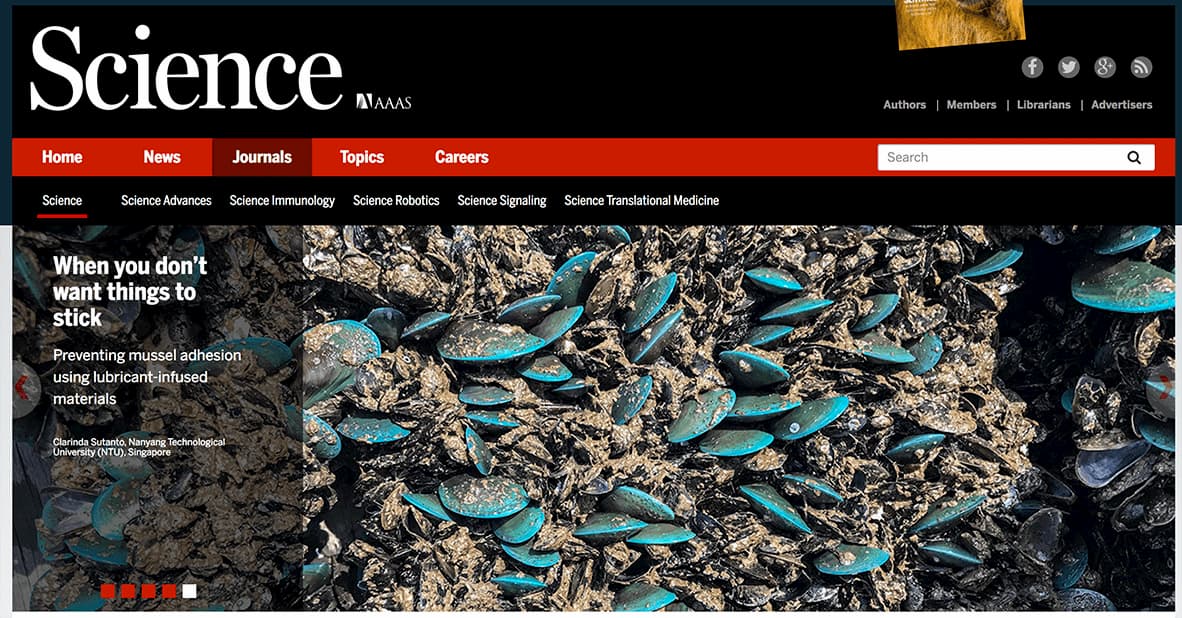This screenshot captures the top section of a "Science" website. In the top left corner, the word "Science" is prominently displayed in large white letters against a black background. Directly beneath this is a red navigation bar featuring options labeled "Home," "News," "Journals," "Topics," and "Careers," with a search bar on the right end. The "Journals" option is highlighted.

Below this red bar is another black navigation bar with categories: "Science," "Science Advances," "Science Immunology," "Science Robotics," "Science Signaling," and "Science Translational Medicine." The "Science" category, the first option, is currently selected.

To the left of the screen, there is a section titled "When You Don't Want Things to Stick: Preventing Muscle Adhesion Using Lubricant-Infused Materials," alongside a photo depicting the ocean floor. The image shows round, turquoise-blue mussel shells emerging from the ground, all pointing upward.

At the top right, the edge of another image is partially visible, displaying a yellow object. Additionally, a series of links are listed, including "Authors," "Members," "Librarians," and "Advertisers," accompanied by icons for Facebook, Twitter, Google Plus, and another social media platform.